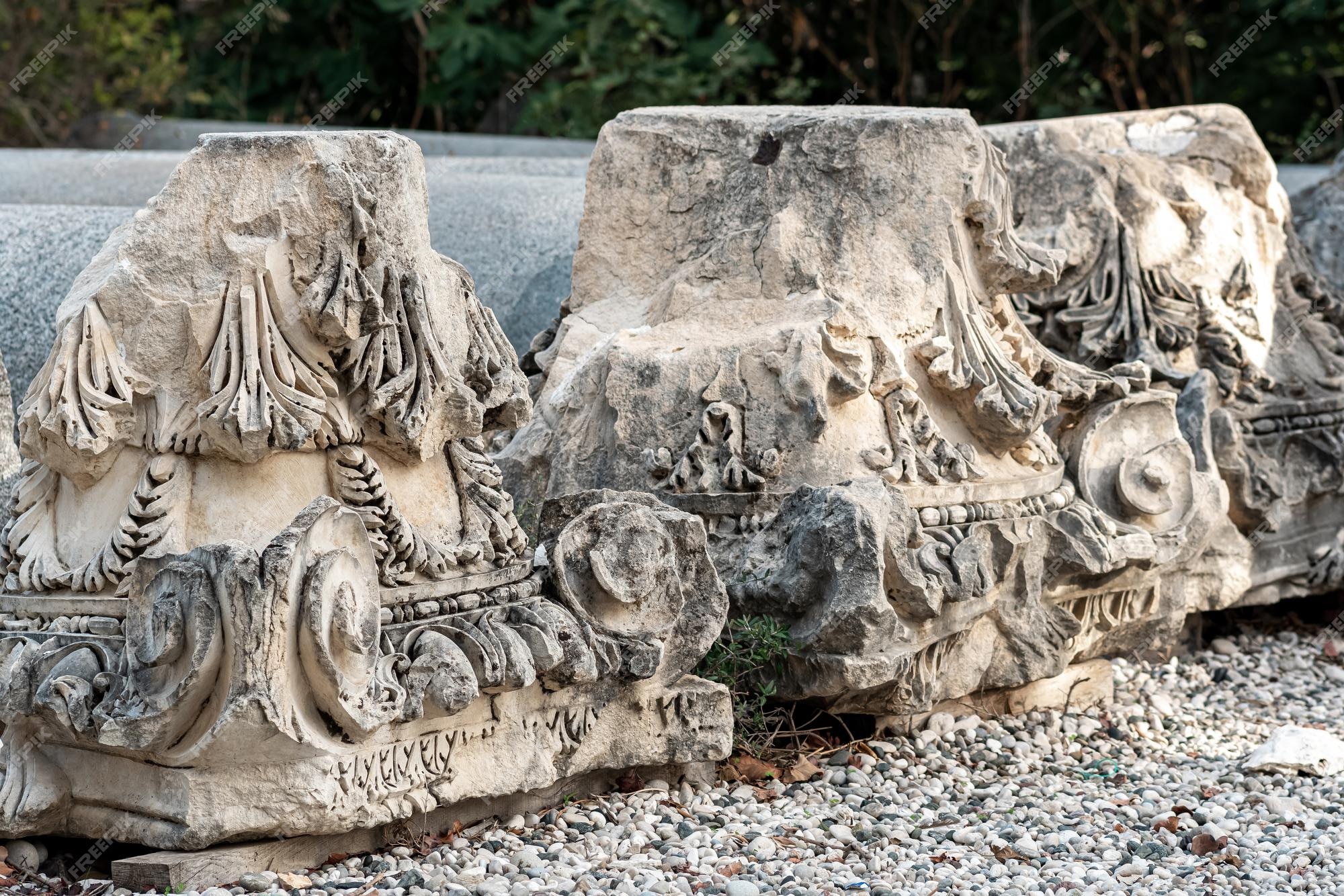This image, taken outdoors in the daytime, captures remnants of three ancient stone carvings, likely from the Greek or Roman era, based on their stylistic features. The stones are predominantly white marble, but time and weather have eroded them, giving them a grayish, sand, and blackish appearance in parts. Each carving features intricate designs, including rope-like swirls and ionic curls, evocative of ancient architectural details. The tops of the structures are smoothed out, resembling folded fabric. The carvings rest on a bed of gray gravel stones, amid some brown rocks, with green trees forming the background. Scattered leaves and patches of grass grow between the rocks, and there’s visible space beneath parts of the stones where something could fit. The words "Free Pick" appear in white capital letters, diagonally across the top left of the image.